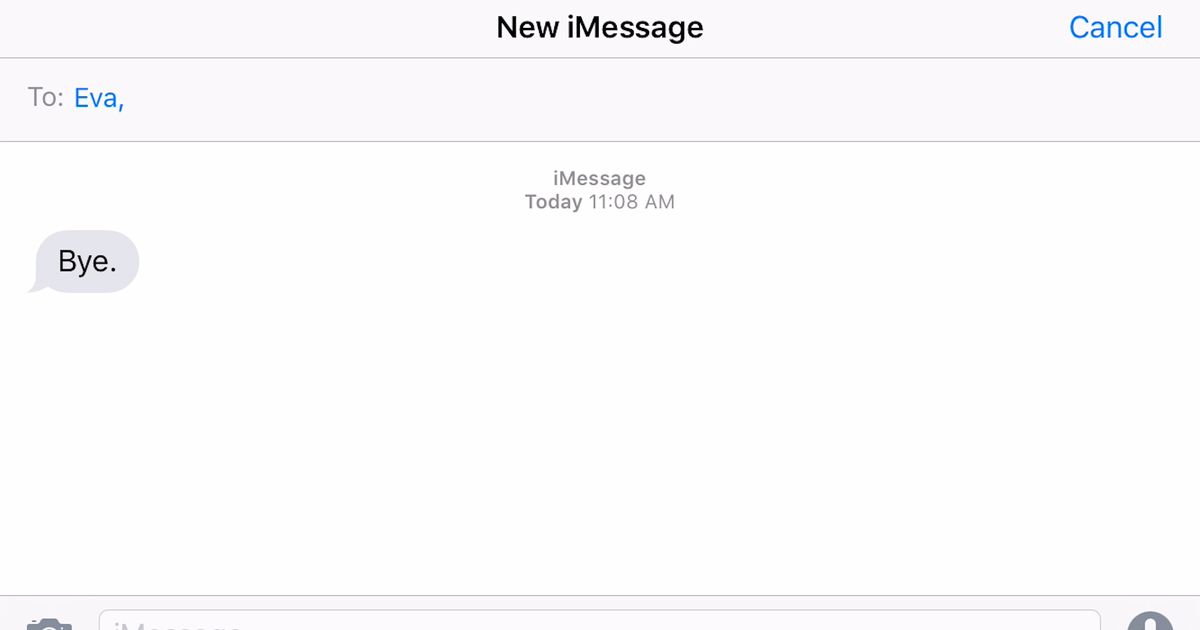This image is a wide, rectangular screenshot of an iMessage interface on a Mac laptop. At the top of the interface, the text "New iMessage" is displayed in black font, with a "Cancel" option in blue font on its right. Below this, on the far left, it says "To:" followed by the recipient's name, "Eva," which is highlighted in a light blue color.

The body of the message occupies a white background. Centered at the top of this section, in grey font, is a timestamp reading "Today, 11:08 AM." Below the timestamp, on the left side of the screen, there is a text message in black font that reads, "Bye, BYE." The image is cropped, revealing only the very top of the message bar at the bottom center, along with the top parts of the camera icon (to the extreme left) and the microphone icon (to the extreme right).